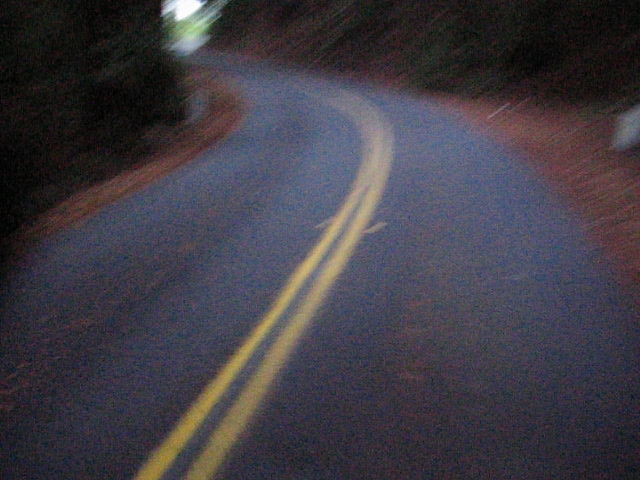This grainy and dark photo captures a winding two-lane mountain road, marked with a solid double yellow line. The scene, viewed from a first-person perspective, is closely cropped and blurry, giving the impression of motion and adding to the sense of speed as the road curves to the left. The asphalt is flanked by dark brown dirt or rocks and dense vegetation that appears almost black. On the left side, more distinct green grass can be seen near the road's edge, while to the right, a gray rock stands out amidst the gloom. The horizon ahead opens up slightly, revealing a patch of clear sky and a hint of bright white and green, possibly indicating open land or vegetative clearing. The surrounding area is dominated by large, dark, possibly vegetation-covered hills lending an imposing presence to the overall moody and dim environment. There are no vehicles or signs of human activity, enhancing the isolated, almost eerie atmosphere of this winding mountain passage.